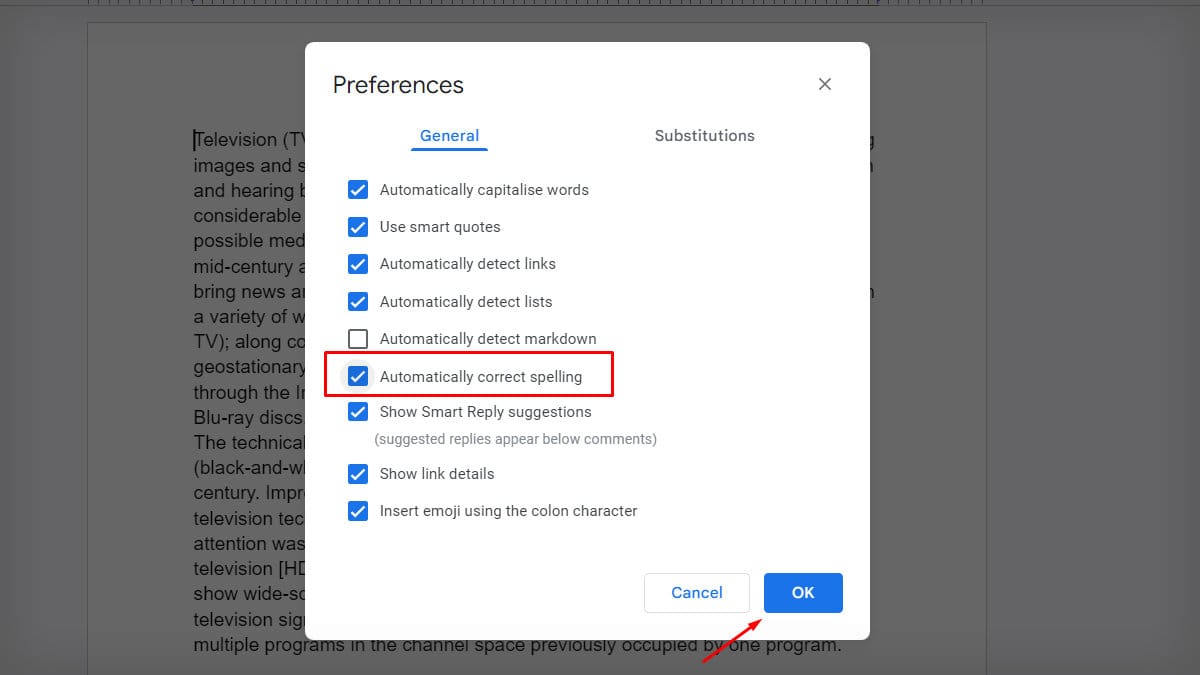The screenshot captures an interface of a reading website or e-reader platform, presented in a horizontal format, suggesting it's displayed on a desktop rather than a tablet or smartphone. The background features text laid out in a single-page format, resembling an article with justified font alignment, though it appears grayed out, keeping the focus on the foreground.

Prominently overlaid on the text is a white pop-up box labeled "Preferences." Within this pop-up, two tabs are visible: "General" and "Substitutions." The "General" tab is highlighted in blue and underlined, indicating it's currently selected. In this menu, the user has deselected the "Automatically Detect Markdown" option, which is the only checkbox without a checkmark next to it. Below the options, there are "Cancel" and "OK" buttons.

The screenshot appears to be an instructional tool, as evidenced by the modifications: a red box around the "Automatically Correct Spelling" option and a red arrow pointing to the "OK" button. These annotations suggest that the screenshot is being used to guide someone through a particular process or setting adjustment on the platform.